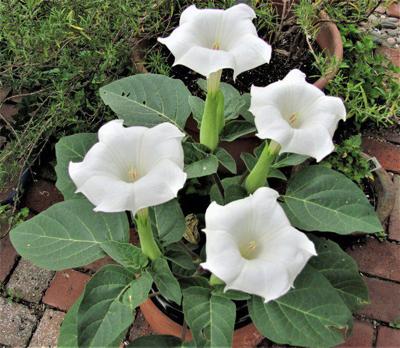The image features a potted datura plant, a relative of the jimson weed, known for its distinctive, large, trumpet-like white flowers. The flowers, four in total, have tips that culminate in sharp points and center with light yellow buds recessed inward. The plant’s stems are a light green, and the velvety, heart-shaped leaves feature thin, light-green veins running through them, resembling an intricate network of veins. These leaves are large and oval, tapering at the ends. The plant is housed in what appears to be a terracotta pot, set on a red brick patio surface. Behind the datura, another vine-type plant in a separate pot can also be seen, adding to the outdoor atmosphere.